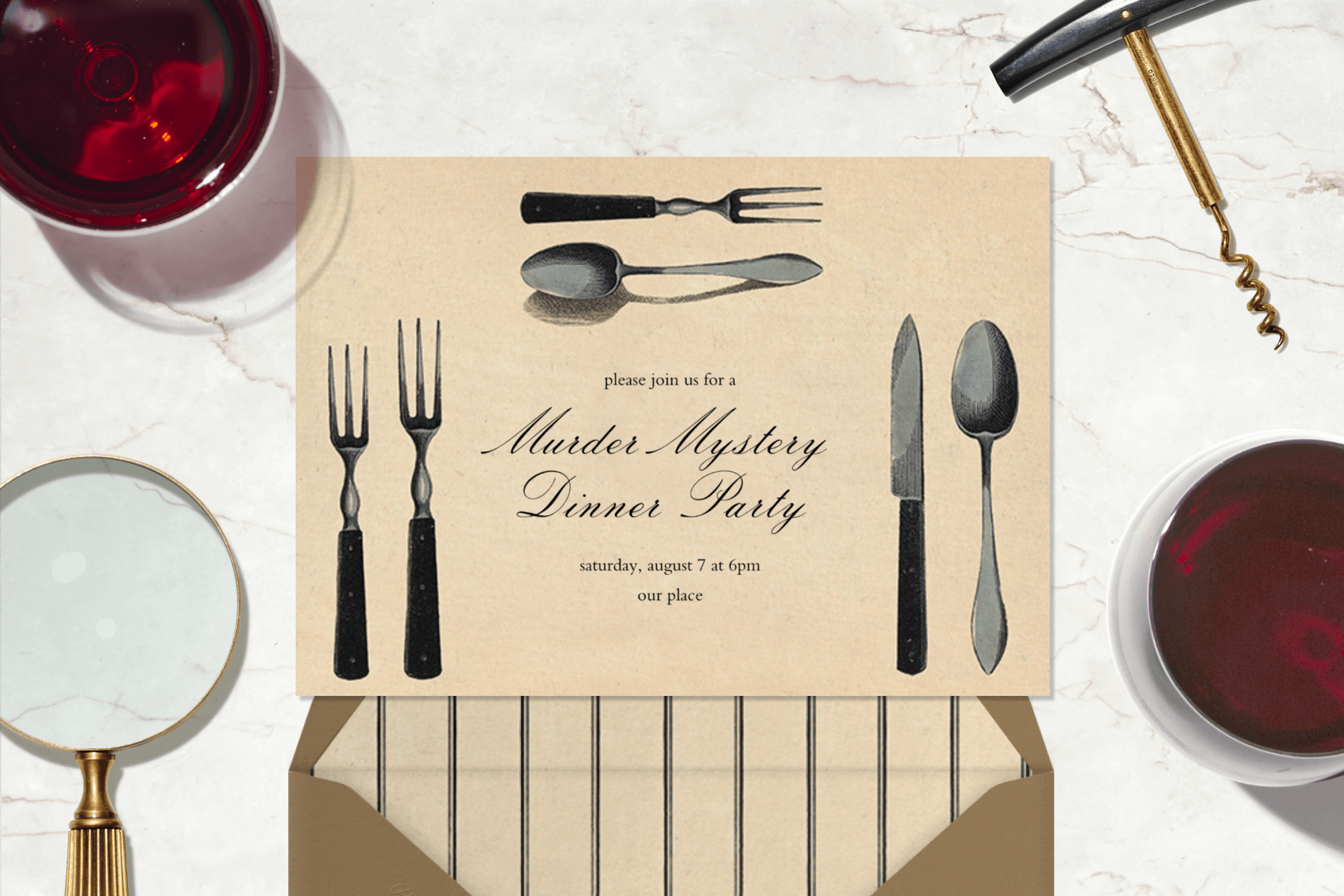The image presents an inviting scene for a murder mystery dinner party. Centered on a white marble table is an off-white greeting card, creatively illustrated with dining utensils. The card reads, "Please join us for a murder mystery dinner party, Saturday, August 7th at 6pm, our place." Surrounding the text are images of dining utensils: two forks on the left side, a fork and a spoon at the top, and a knife and spoon on the right. Below the card is its brown, open envelope. To the left of the card, a gold magnifying glass rests on the table, while two jars with red lids are positioned on the top left and right sides of the card.